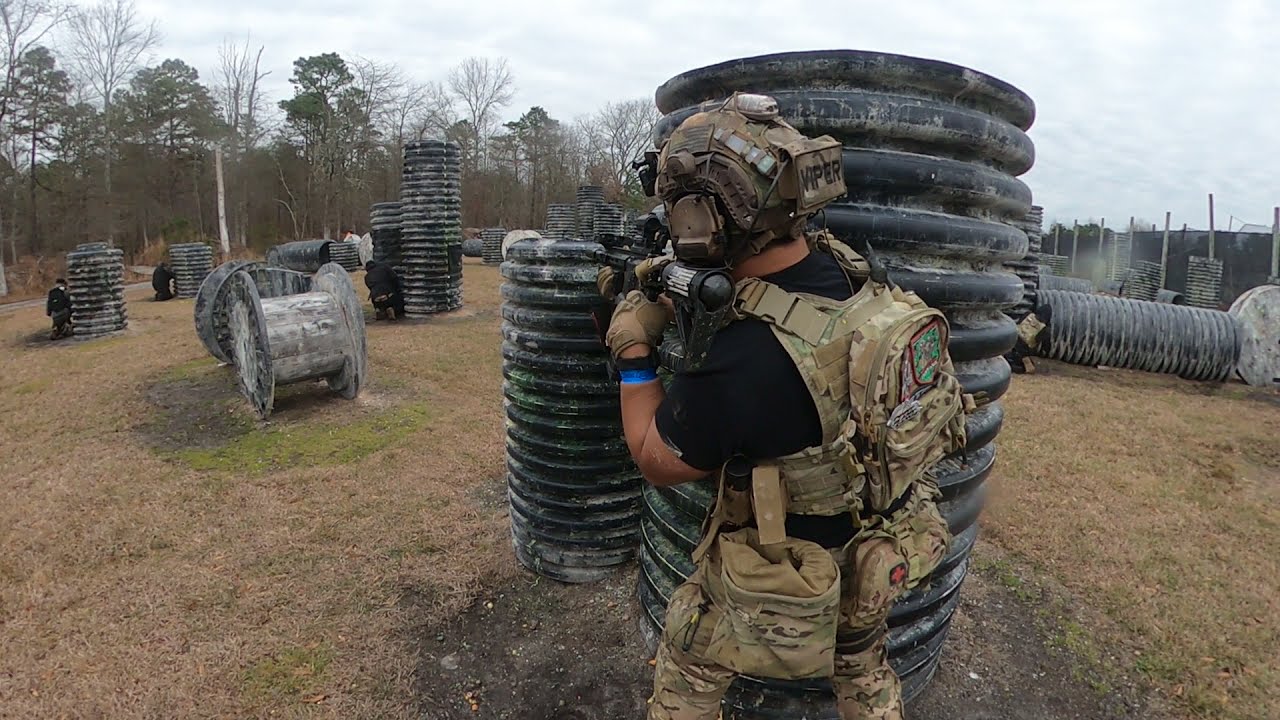In this outdoor photograph, the scene is set in a rectangular, training ground area under a gray, overcast sky. The grass is mostly brown and crunchy, suggesting the time of year is either early winter or early spring. Central to the image is a soldier dressed in full military fatigues, including a helmet, camouflage pants, a black t-shirt, wristbands on his left arm, gloves, and a backpack with various sacks attached to his waist. The soldier’s profile is partially visible as he stands behind tubular equipment, appearing to scout or take cover, possibly pointing a weapon at unseen individuals. The field is dotted with multiple obstacles, including standing and fallen cylindrical objects that resemble plastic tubes, and wooden wire holders, creating an environment akin to a military training session. Other soldiers can be seen crouching and peering from behind these barriers, enhancing the impression that this is a simulated combat or training exercise. In the background, trees frame the scene, emphasizing the outdoor setting.